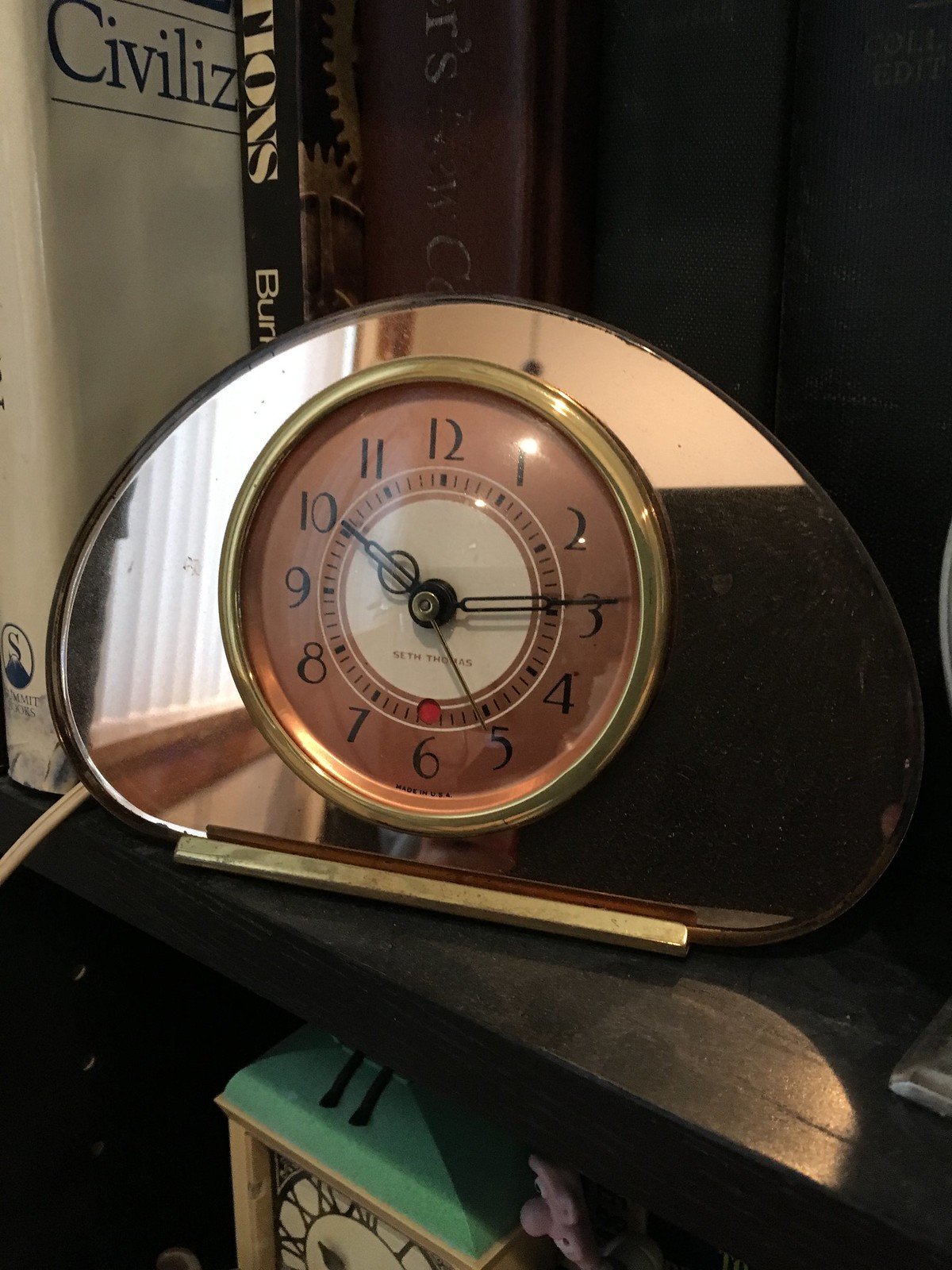The photograph captures a detailed scene centered around a copper-colored, metal clock positioned on a black, adjustable shelving unit. The clock, which is approximately oval-shaped with a flat bottom, features a shiny gold rim and a circular face. The face has a gradient that shifts from a rusty brown outer ring to a pinkish area, and then to a white center where black numbers and clock hands mark the time at 10:15. Behind the clock, several books are visible, including one with the title partially obscured, reading "CIVILIZ," presumably "Civilization." The shelf is part of a modular unit, and in the bottom portion of the image, another clock is visible—this one featuring Roman numerals and a square or rectangular shape with a green top.